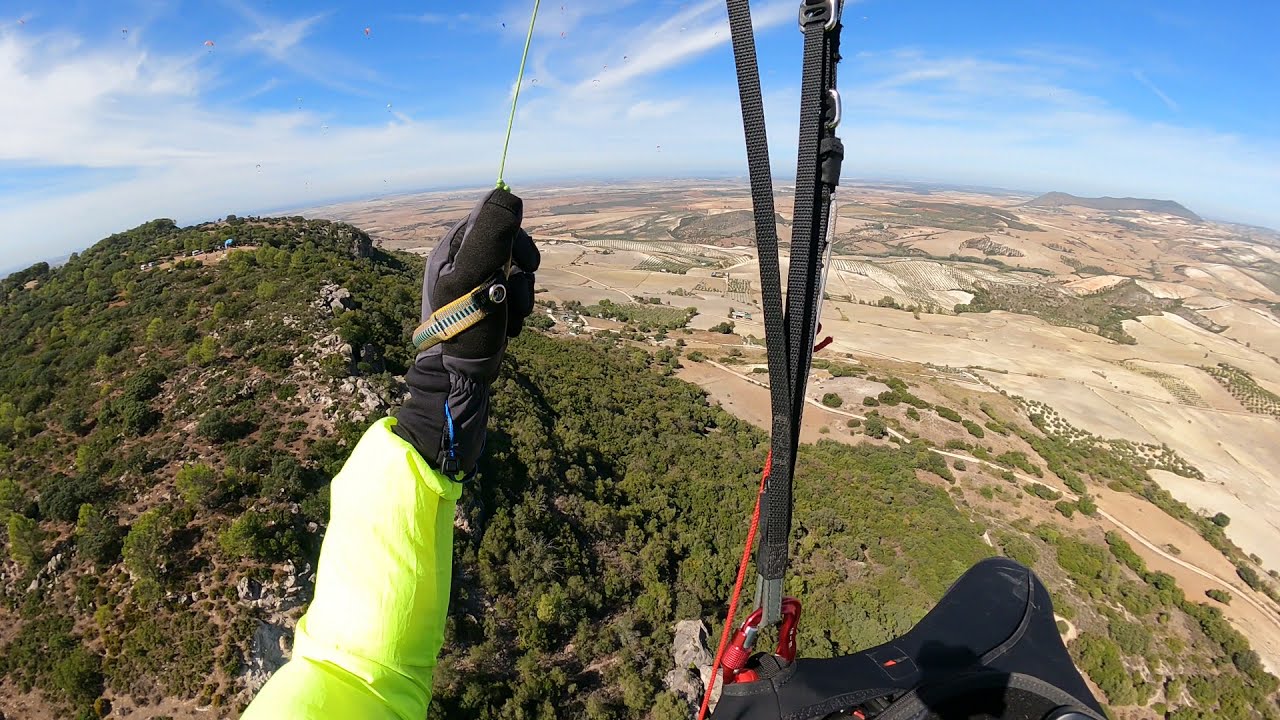The image captures an exhilarating moment from an aerial perspective, likely taken with a GoPro camera, providing a sweeping view of the landscape below. The person appears to be hang gliding or parachuting, with their left hand prominent in the frame. The hand is clad in a black and gray glove, gripping a paracord that runs vertically. The individual's arm, covered in a neon green long-sleeve shirt reflecting light, extends from the elbow to the wrist where it meets the glove. Additional equipment includes black straps, some featuring red clamps, and a red bungee cord hanging from them.

From this lofty vantage point atop a mountain, the viewer can see a diverse landscape. The foreground reveals a rocky terrain with some short shrubs and a discernible line of rocks. In the bottom right corner, a pipeline runs from the right towards the center, descending into a distant village. The midground and background of the image are predominantly brown, indicative of a desert-like environment, interspersed occasionally with parcels of farmland and sparse vegetation.

The land appears curved due to the camera lens distortion, creating an exaggerated horizon. The sky above is a bright blue, decorated with sporadic light clouds. Various colors dominate the scene, including multiple shades of green, brown, orange, and tan in the landscape, while the vibrant neon of the parachuter’s sleeve stands out. This image, set outdoors in the middle of the day, captures both the thrill of extreme sports and the expanse of natural beauty below.